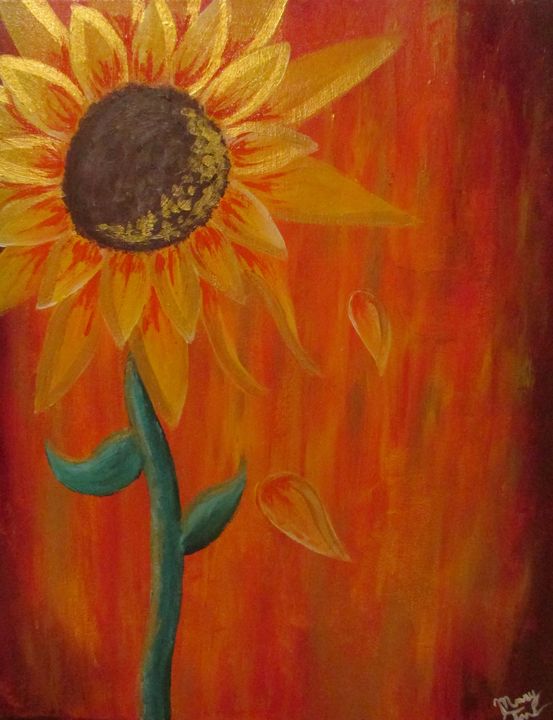The image depicts an oil painting centered on a vibrant sunflower rising from a green stem, with two symmetrical leaves branching out. The sunflower boasts two concentric layers of petals: an inner row of smaller yellow petals and an outer row of larger ones. The flower's circular center is brown, adorned with yellow pollen dots, particularly noticeable on the right side. Radiant reddish hues accentuate the petals, adding depth to the painting.

The sunflower is set against a reddish-yellow background that darkens towards the edges, especially the top right and bottom right corners. The background seamlessly blends with the colors of the falling petals, which cascade downward from the flower, contributing to a sense of movement within the piece. In the bottom right corner, partially cut off, is a small white signature, likely that of the artist.